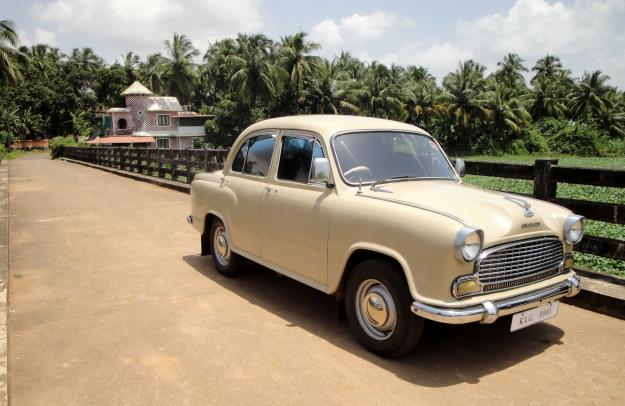This detailed photograph captures a classic, old-fashioned car from the 1930s or 40s, positioned on a beige roadway in what appears to be a tropical setting. The car, a light pinkish-yellow or tan color, features distinctive chrome accents including the wheels, hubcaps, and ornate round headlights. The steering wheel is on the right-hand side, and the vehicle has four doors with darkened side windows.

Adjacent to the car is a wooden fence, extending towards a house in the background. The house has a structure reminiscent of an island dwelling with red and white siding, giving it a somewhat modern yet tropical architectural feel. Surrounding the house are numerous, dense palm trees with large, green fronds. The setting includes a light brown cement driveway leading up to the house, and patches of grass can be seen between the fence and the palm trees. The sky overhead is a bright, sunlit expanse with some clouds, emphasizing the warm, island-like ambiance.